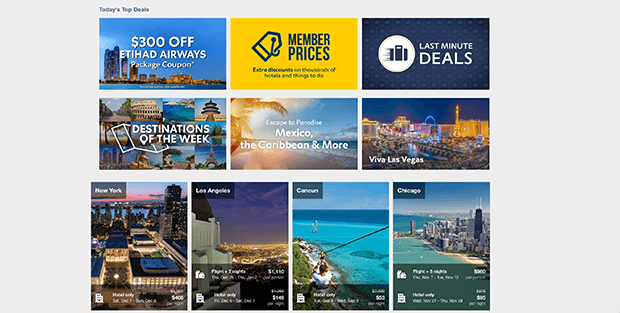In the image titled "Today's Top Deals," the top section features six enticing offers. The top left deal advertises "$300 off Etihad Airways package coupons," displayed in white text. The center top offer reads "Member Prices, Extra Discount" in blue text on a yellow background. The top right showcases "Last Minute Deals," with white text on a blue background. Moving to the lower half of the top section, the bottom left deal highlights "Destinations of the Week" in white text against a scenic ocean backdrop with trees, featuring destinations from Europe to paradise, Mexico to the Caribbean, and more. The bottom center presents "Europe to Paradise," also in white text on a similar oceanic background. Lastly, the bottom right corner displays "Viva Las Vegas," written in white with a background of Las Vegas city lights.

The lower section of the image presents four additional deals. Starting from the left, there is an offer for New York, depicted with a nighttime cityscape of buildings. To its right, there is a deal for Los Angeles, illustrated with a building and city lights. Further right is an offer for Cameroon, featuring an image of people ziplining. Finally, the bottom right corner showcases Chicago, set against a backdrop of the city's skyline with buildings and an ocean.